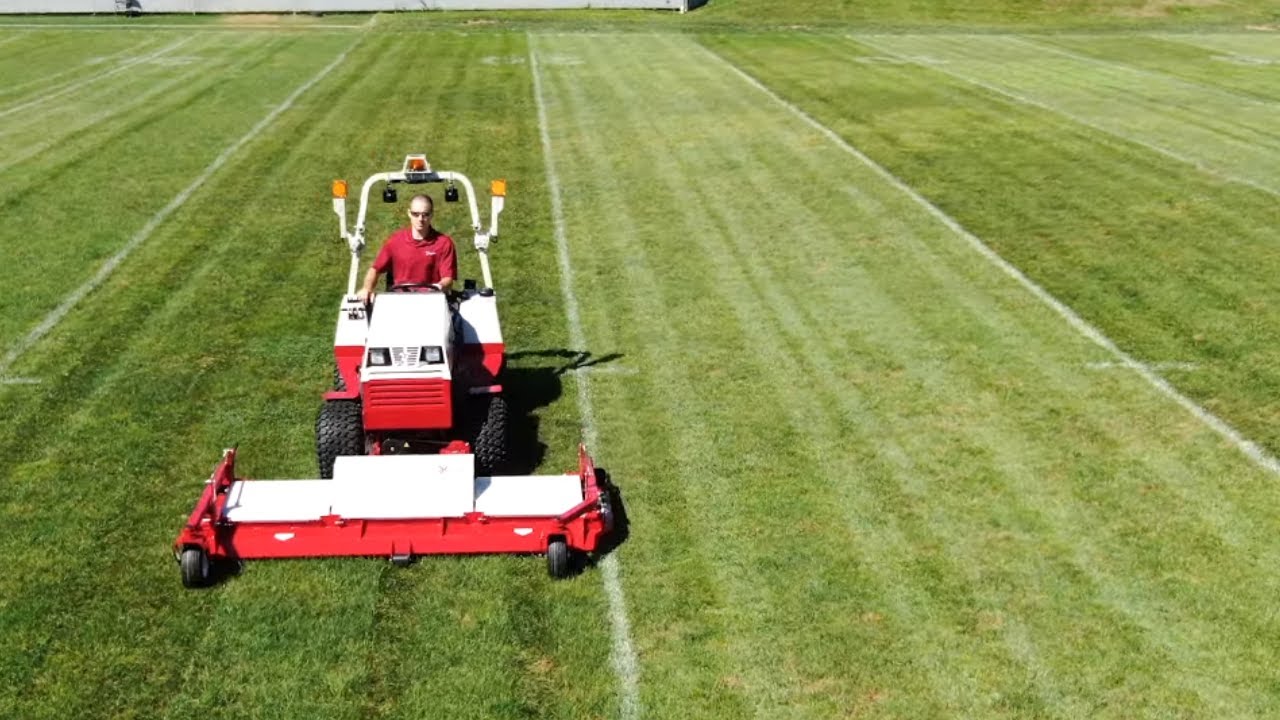A large green grass field, likely an American football field, stretches out with clearly marked lines in five-yard increments and numbers visible in the background. At the forefront, a sizable lawnmower with a white body and red bottom is actively working to meticulously shape the field. This mower is being operated by a man in a red shirt and sunglasses, who sits prominently on the left side of the image. The man is white and appears focused as the mower's front blades trim the grass. The rows created by the mower are perfectly aligned, adding to the overall precision and maintenance of the athletic field.